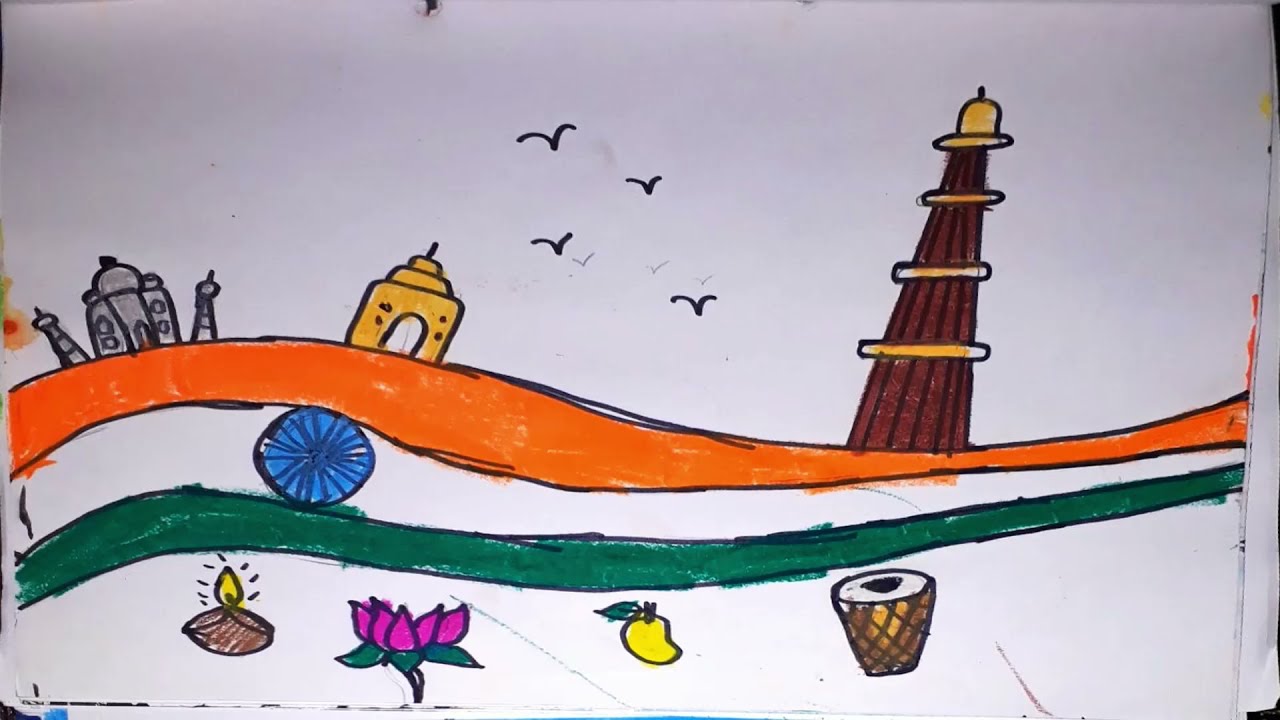The image is a child's drawing on a white canvas, featuring a series of simple and vibrant elements. In the foreground, there is a tricolored flag spanning horizontally with orange at the top, white in the middle, and green at the bottom, resembling the flag of India. A blue circle with light gray spokes is situated in the center of the white stripe, enhancing the flag's likeness to the Indian national flag. 

Above the flag, in the top section of the image, there are three prominent structures. To the left, a gray castle is depicted, followed by a yellow castle in the middle, and a tall brown and yellow tower to the right. This tower has a bell-shaped top with gold bands encircling the structure. In the background, a smudged gray area appears, possibly representing clouds, with rudimentary black birds flying in the sky drawn as small curved V's, reminiscent of seagulls.

Below the flag, four distinct objects are illustrated. From left to right, they include a yellow flame on a brown circle, a pink lotus blossom on a green lily pad, a yellow pear, and a cut piece of ham. Additionally, a green wavy line with a black outline separates these objects from the flag, adding a whimsical touch to the child's imaginative creation.